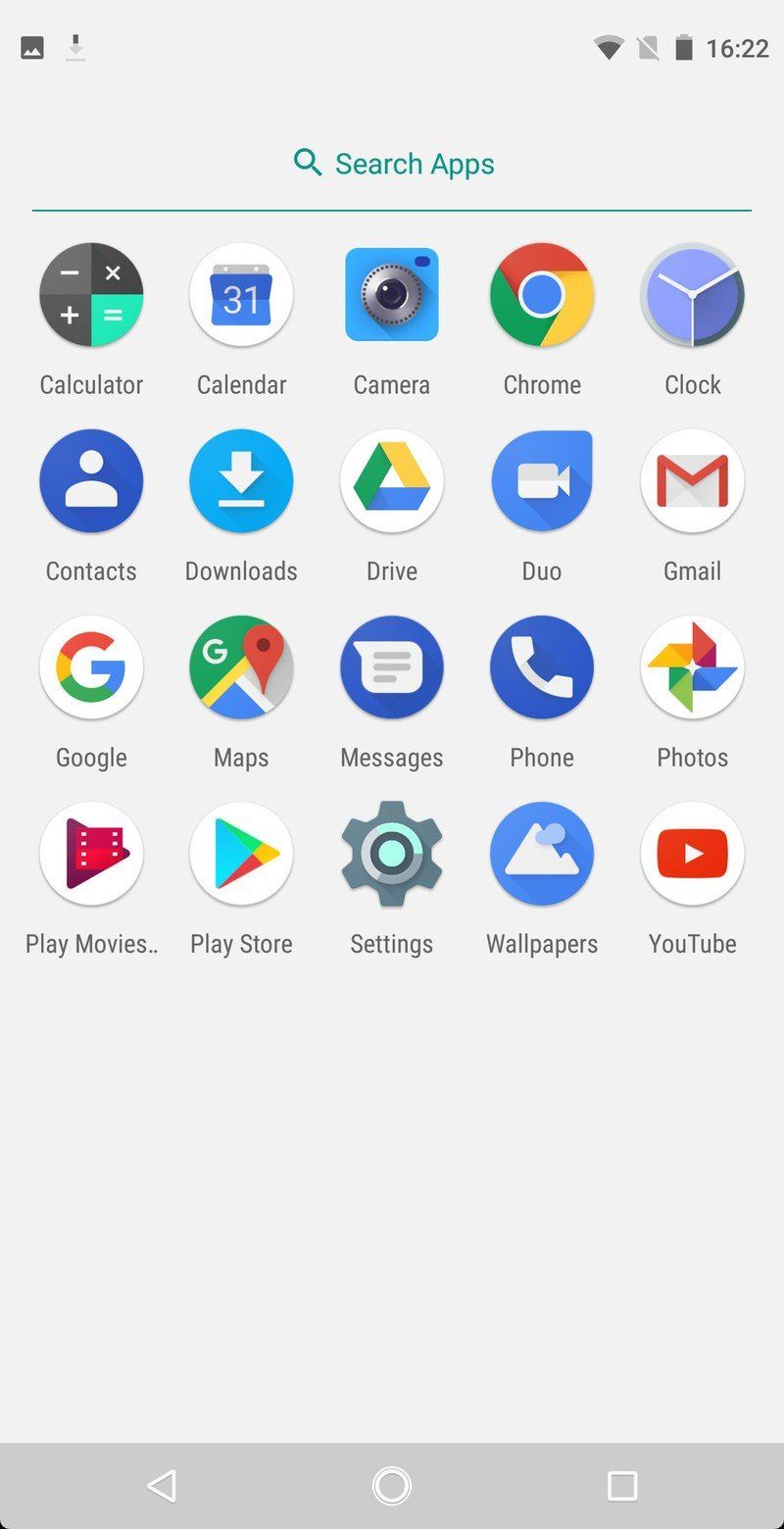The image depicts the home screen of a smartphone, primarily designed with a green theme. At the top, there is a green magnifying glass icon next to the text "Search apps," followed by a long green horizontal line underneath. Below this line, there is a circular icon featuring an X, a plus sign, and an equal sign, resembling a calculator.

The home screen displays a grid of app icons arranged in rows:

- **First Row**: Calendar, Camera, Chrome, and Clock.
- **Second Row**: Contacts, Downloads, Drive, Duo, and Gmail.
- **Third Row**: Google Maps, Messages, Phone, and Photos.
- **Fourth Row**: Play Movies, Play Store, Settings, Wallpapers, and YouTube.

The YouTube icon is a distinctive red square with a white play arrow pointing towards the right.

In the upper right corner of the screen, the battery icon is fully charged, and the current time is displayed as 16:22.

At the bottom of the screen, there's a gray navigation bar. This bar includes three icons: a circle representing the Home button, an arrow pointing to the left for the Back function, and a square for accessing recent apps.